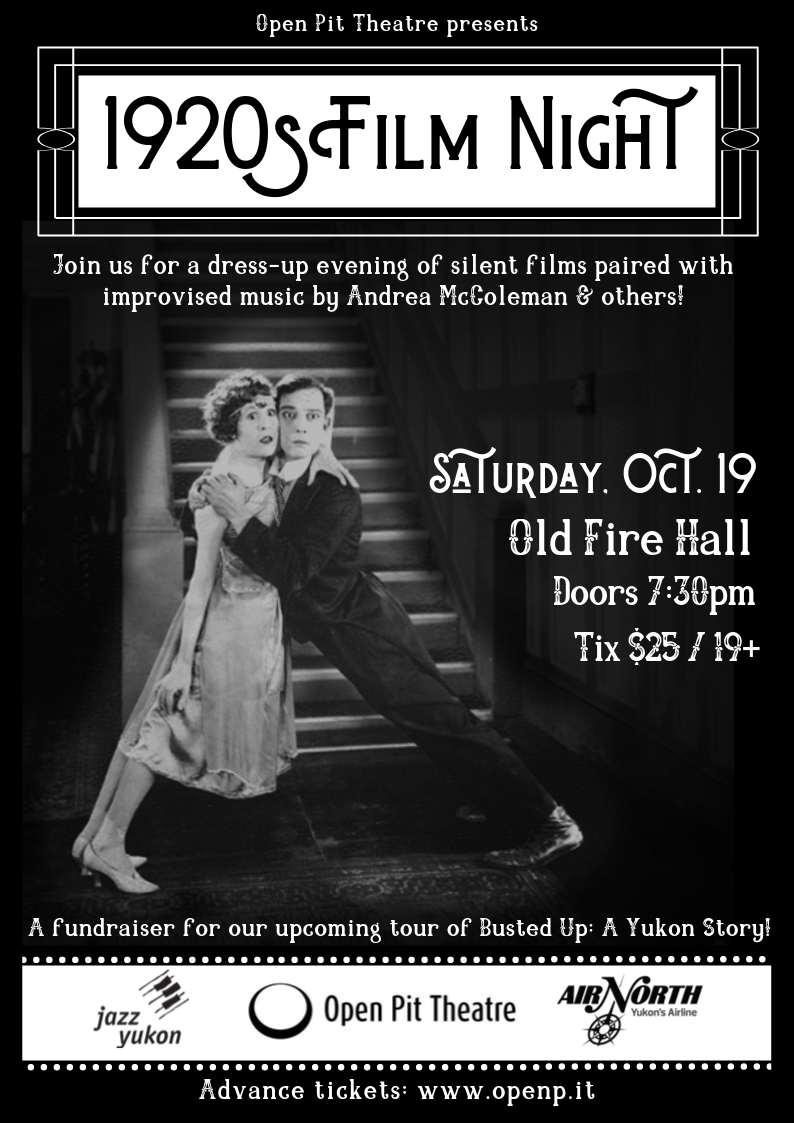The poster has a predominantly black background with multiple sections of text and an image. At the top, it reads "Open Pit Theater Presents" in white text. Below this, a white bar contains the text "1920s Film Night" in black. Following this, in smaller white text, it invites viewers to "Join us for a dress-up evening of silent films paired with improvised music by Andrea McColman and others."

Central to the poster is a black-and-white photograph depicting a man and a woman standing in front of a staircase. The woman is on the left and appears to be standing on her tiptoes while leaning towards the man. The man, positioned on the right, mirrors her pose, balancing on his toes and leaning toward her. Both are looking into the camera with an expression of apprehension.

To the right of the image, white text lists event details: "Saturday, October 19th, Old Fire Hall, Doors 7:30 PM, Tix $25/19+."

At the bottom, in white text, it mentions: "A Fundraiser for our Upcoming Tour of Busted Up, a Yukon Story." Beneath this, a white bar contains logos and names "Jazz Yukon, Open Pit Theater, Air North," followed by the URL for advanced tickets: "www.openp.it."